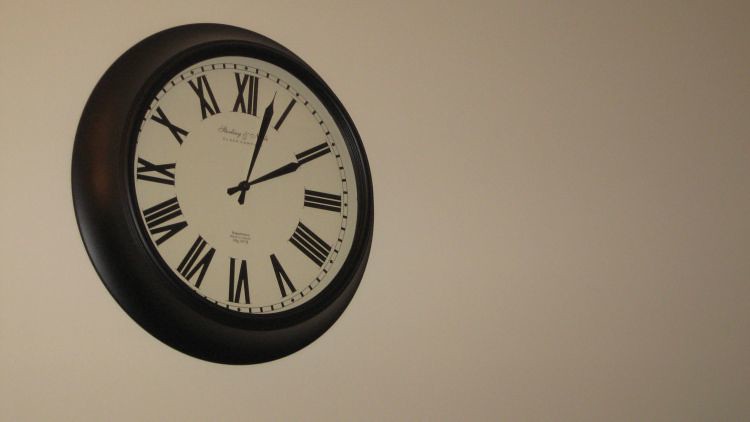The image features a beautifully decorated wall painted in a light orchid shade. Dominating the scene is a large, round clock mounted on the wall. The clock is encased in a very dark brown frame, almost black in appearance, and has a prominent white face. The time displayed is approximately four minutes past two, indicated by sleek black hands. Surrounding the clock face are elegant black Roman numerals marking the hours. Beneath the twelve and just above the six, subtle inscriptions can be discerned, adding a touch of sophistication to the design. The clock is notable for its substantial thickness and is protected by a gleaming glass cover, enhancing its classic and refined look.